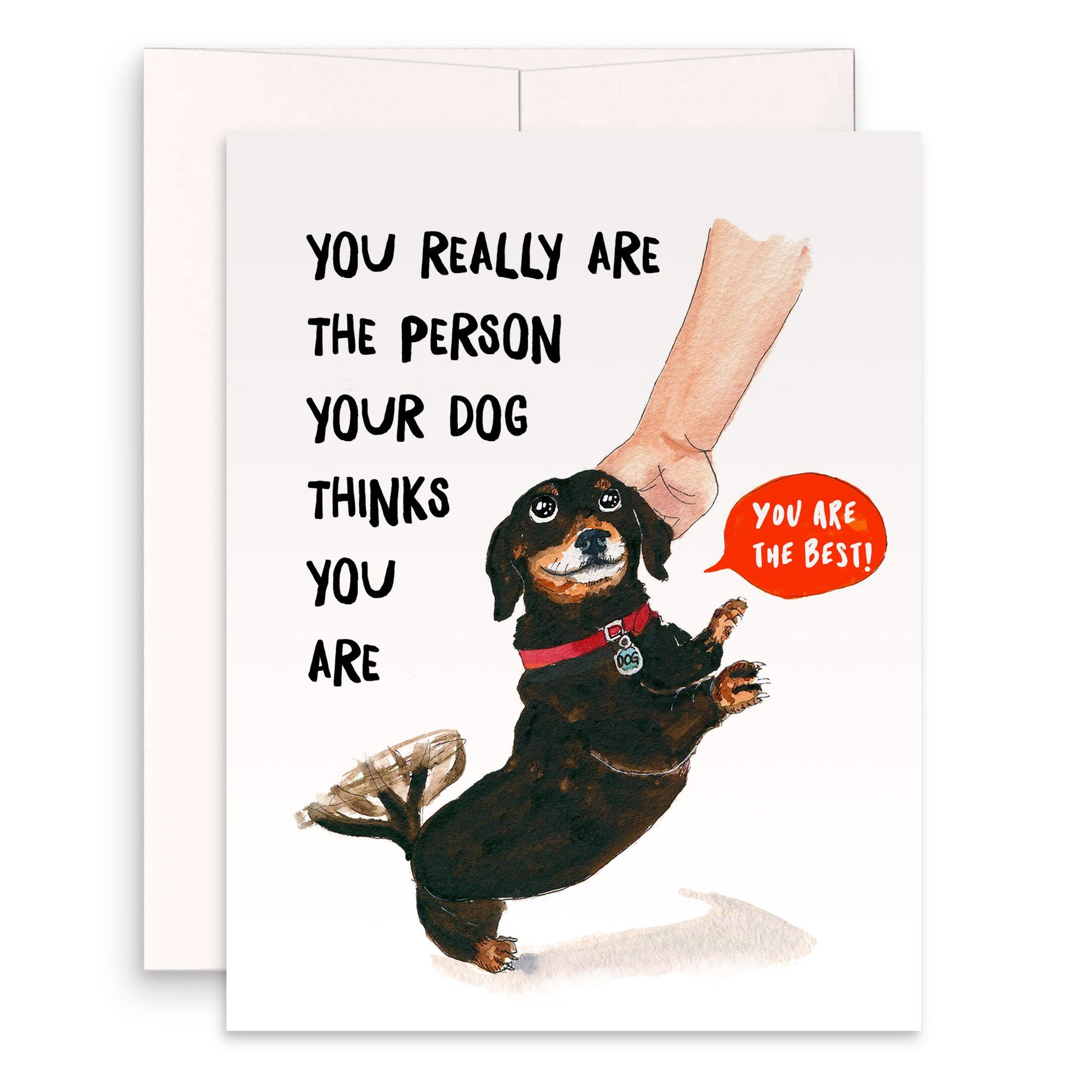The image features a greeting card displayed against a plain white background with a white envelope partially visible behind it. The card itself is vertically oriented, akin to a standard 9.5 x 11 sheet, and has a white front adorned with black text that reads, "You really are the person your dog thinks you are." To the right of this text, there is an illustration of a small dog, likely a chihuahua or dachshund, with a dark brown body, light brown snout, and white around its mouth. The dog has large, endearing eyes and is wearing a red collar with a tag labeled "dog." The dog appears to be excited, with its tail wagging energetically, as it looks up at an outstretched hand reaching down from the upper right of the card to pet it. This hand seems to belong to a Caucasian person. Additionally, a red speech bubble near the dog contains the text, "You are the best," printed in white. The overall scene is heartwarming and playful, capturing the affectionate bond between a pet and its owner.